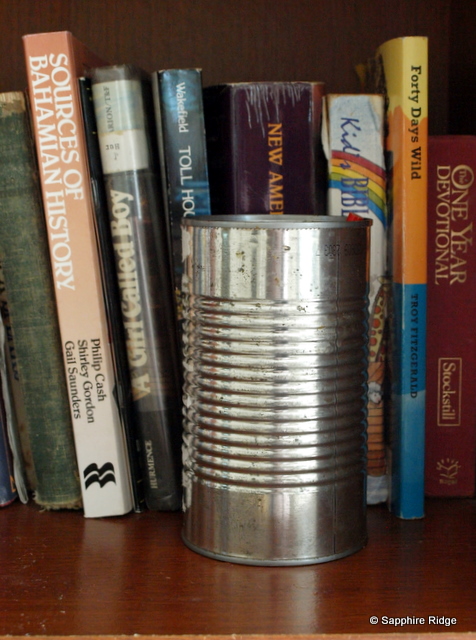A carefully arranged photograph showcases a metallic can positioned in front of a diverse collection of standing books on a wooden bookshelf. The books, varying in size and shape, appear to be older volumes possibly from the 1980s and 1990s, adding a nostalgic touch to the scene. Among the visible titles are "Sources of Bahamian History" by Philip Cash, Shirley Gordon, and Gail Saunders, and "A Girl Called Boy," though the author's name is difficult to discern. Another identifiable book is by an author named Wakefield, titled "Toll Hook Something." Additional titles include "New A.M.E." or perhaps "New America," "Kid's Bible," "Forty Days Wild," and "One Year Devotional." In the bottom right corner, a copyright mark for Sapphire Ridge is visible. The presence of the metallic can in front of these books adds an intriguing element, possibly suggesting that the photo was taken by those credited with the copyright.